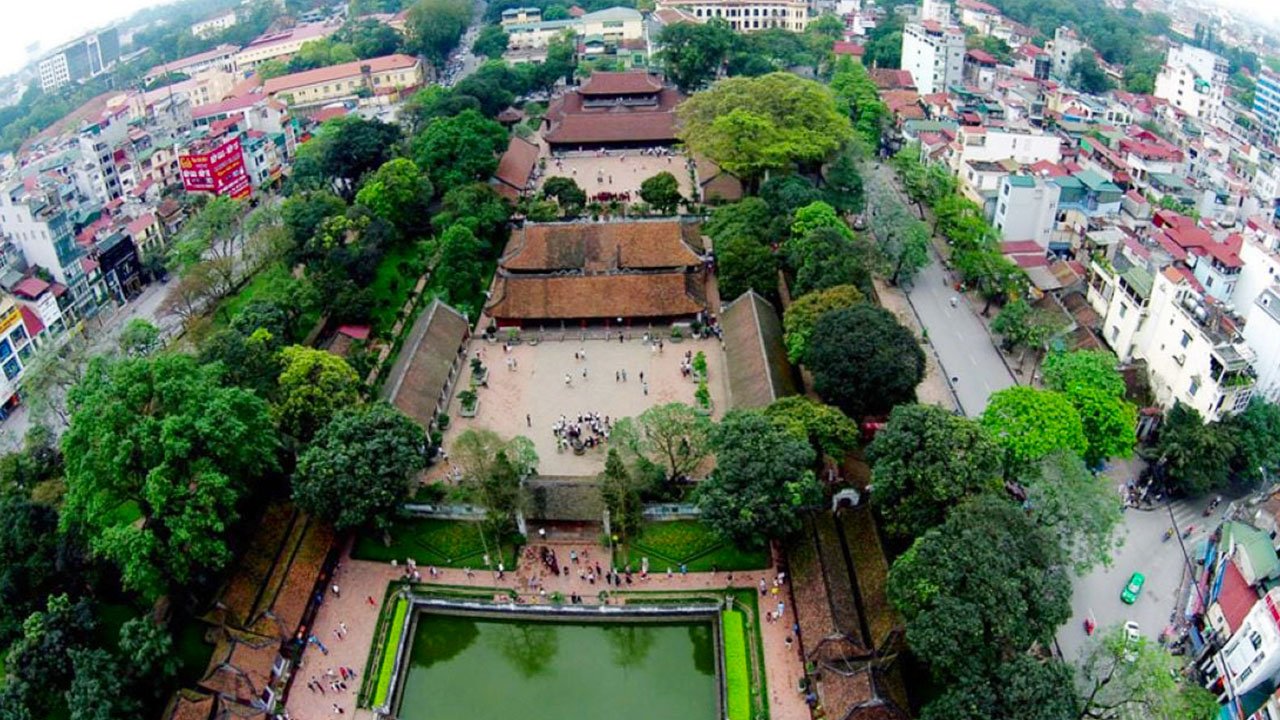This detailed overhead aerial photo, likely taken with a high-end drone, showcases a vibrant cityscape centered around a distinctive park. Dominating the scene is a man-made square water feature, tinged green and reflecting nearby trees, surrounded by walkways with people milling about like tiny ants. The park features a variety of vividly colored and dense treetops, from dark nearly black hues to vibrant greens and yellows, giving a striking contrast. Amidst this verdant sanctuary, sandy paths meander, leading to several low buildings with brown roofs.

To the left and right of the park, the city unfolds with a plethora of buildings in diverse styles and colors, including red, brown, white, and even pink roofs. Streets and side roads weave through the urban landscape, populated with vehicles and bustling human activity. The layout suggests a public garden or a recreational area at the center of this urban environment, making the image a panoramic capture of a serene green oasis amidst the city’s architectural diversity.